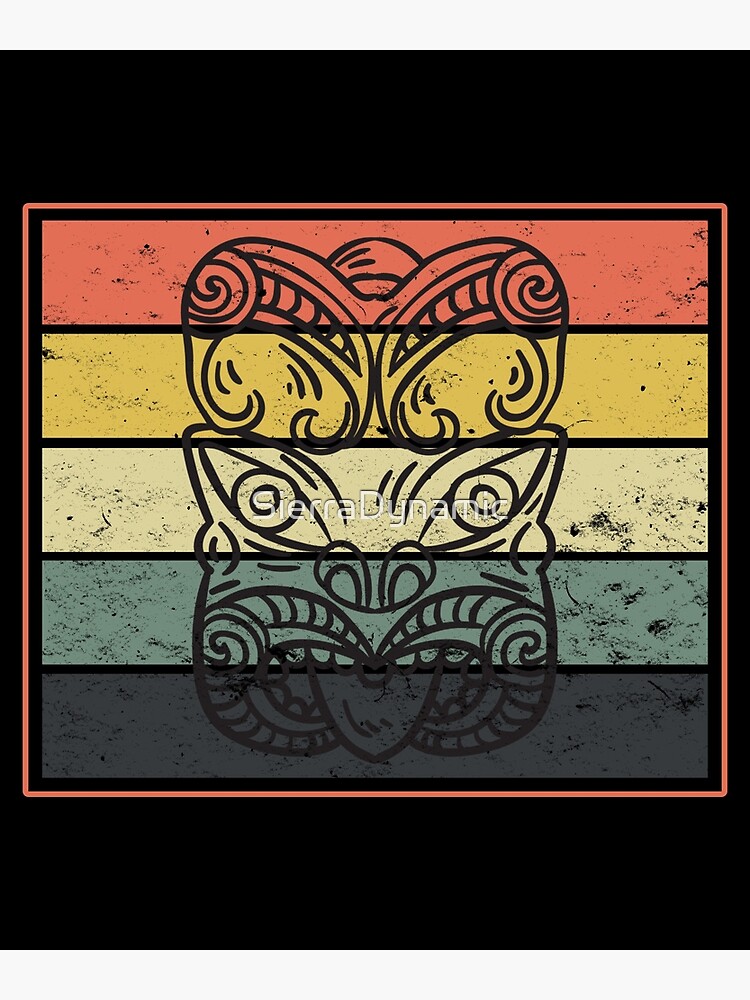The image features a digital drawing set against a pure black background with a large orange square outline encasing the entire composition. Just inside this orange outline is a black border. Within this bordered square, there are five horizontal stripes of color, arranged from top to bottom as red, yellow, white, teal, and gray. A detailed, swirling line drawing of an Asian-inspired dragon spreads across all the colored stripes, crafted with intricate curves and spirals. This dragon design includes prominent features such as eyes, teeth, and potentially a tongue, giving it an expressive, almost mythical appearance. In the center of the white stripe, the words "SierraDynamic" are inscribed with a capitalized "SND" and no spaces, hinting that it might be a logo. This amalgamation of colors, patterns, and the elaborate dragon design evokes a striking and vibrant aesthetic.